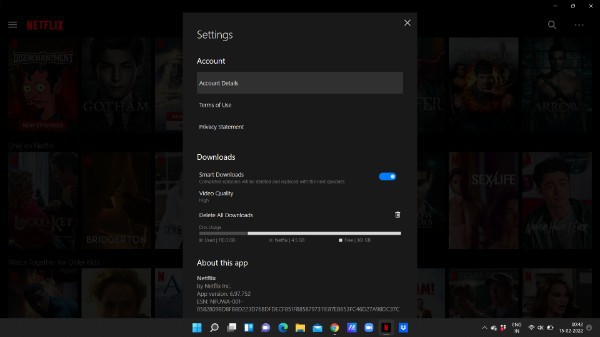This screenshot captures the Netflix website as viewed on a desktop device, with an active pop-up menu overlaying the main interface. The background of the website is subtly visible through a dark, semi-transparent filter, while the pop-up menu stands out in a lighter shade of black. In the top-left corner, the iconic Netflix logo is prominently displayed in bold red font, adjacent to a drop-down menu symbolized by three vertically aligned white horizontal lines. Below the header, three rows of indistinguishable movie and show thumbnails are partially obscured by the dark overlay. 

At the center of the screen, a pop-up menu labeled "Settings" in white font commands attention. On the upper right corner of this menu, there is a small "X" icon for closing the dialogue box. The settings menu lists several options: "Account," followed by an unreadable text, and “Terms of” followed by additional indistinct text. Further down, there is a section titled "Downloads" with an option for "Smart Downloads," which is currently activated, indicated by a blue toggle switch. Lastly, the menu displays "Video Clarity" set to "High," suggesting a user preference for streaming content in the best available resolution.